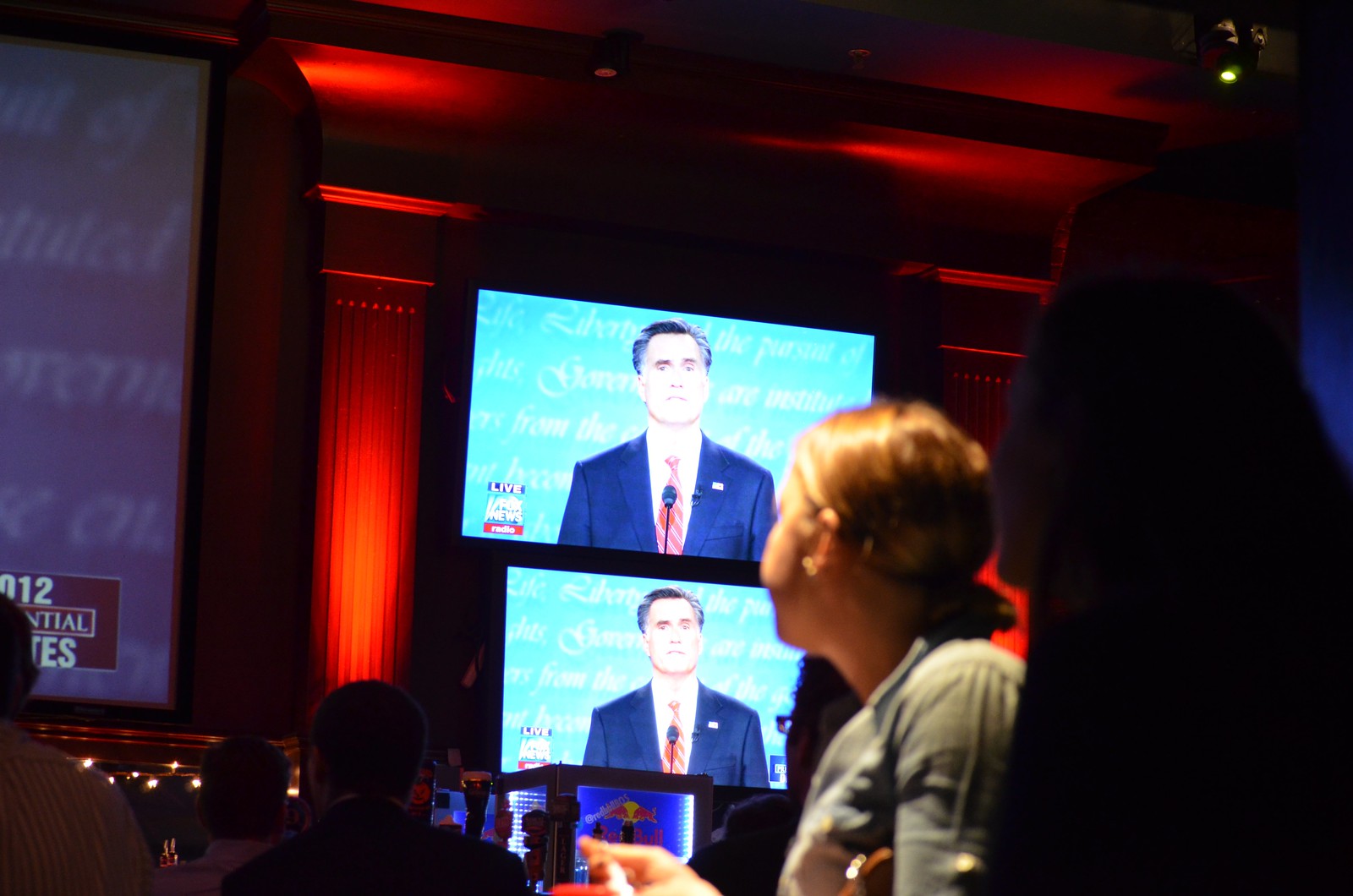The image captures an indoor scene within a large, high-ceilinged convention hall or theater, where a group of attendees is focused on two jumbo screens displaying a live broadcast. Dominating the screens is Mitt Romney, identifiable by his distinctive gray hair, dressed in a black suit, red tie, and American flag pin. Accompanying text indicates that he is speaking live on Fox News Radio, likely during the 2012 presidential campaign. The background of the hall is dramatically lit with red accent lights, enhancing the presentation area against the dark surroundings. In the foreground, a blonde Caucasian woman in a gray t-shirt is visible, seated and turned towards the screens, intently watching the broadcast. Other seated attendees, some partially visible, also direct their attention to the screens, reinforcing the atmosphere of a focused, conference-like environment.